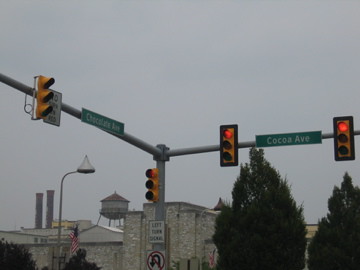A daytime photograph captures a slightly dark, overcast scene at the intersection of Cocoa Avenue and Chocolate Avenue. Naturally lit by the diffused sunlight filtering through thick clouds, the image prominently displays silver-metal traffic lights with yellow signal heads and poles stretching across both sides of the intersection. The traffic lights on Cocoa Avenue show red signals, while the lights on Chocolate Avenue are not visible. Road signs at the intersection indicate "Left Turn Only" and "No U-Turn." In the background, the urban landscape features gray brick or stone buildings, a set of industrial smokestacks, and a water tower. Additionally, two lush green trees add a touch of nature to the scene.